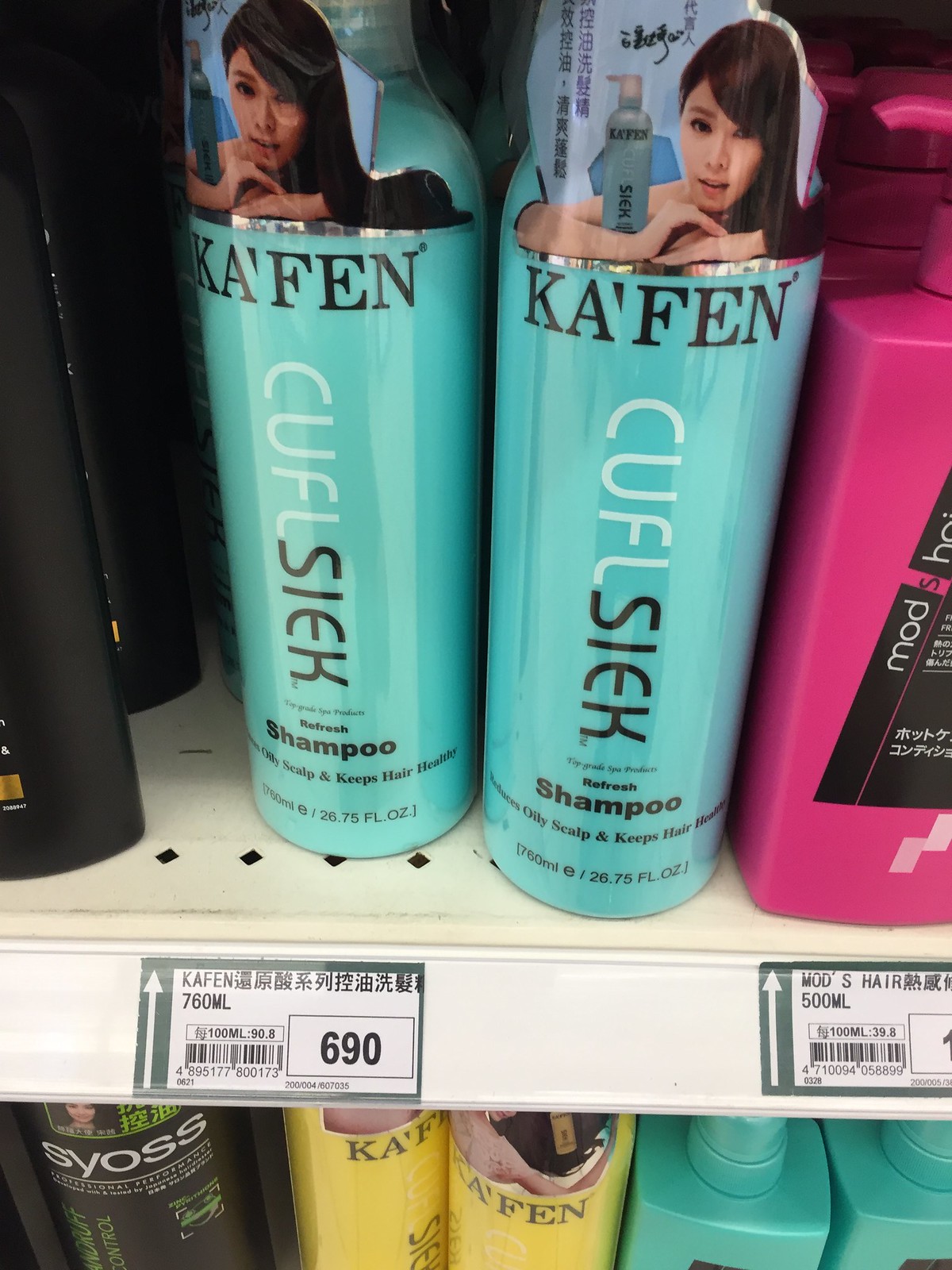This is a detailed photograph taken inside an Asian supermarket, capturing a store shelf lined with various hair products, primarily focusing on two turquoise, tubular bottles of shampoo. The prominent bottles are marked with the brand name "Ká'fèn" spelled in bold black text at the top, alongside a mixture of blue, black, and white text. An image of an Asian woman with long brown hair, cradling the bottle, is prominently displayed on each bottle. The label also includes the phrase "Curl Siek Refresh Shampoo" and indicates that it reduces oily scalp and keeps hair healthy. The product information is rendered in both English and Asian characters. Additionally, a barcode on the shelf signifies a volume of 760 ml for the bottles. Flanking the featured shampoos are other hair products, including ones in pink bottles, indicating the diversity of the offerings tailored for the Chinese market.